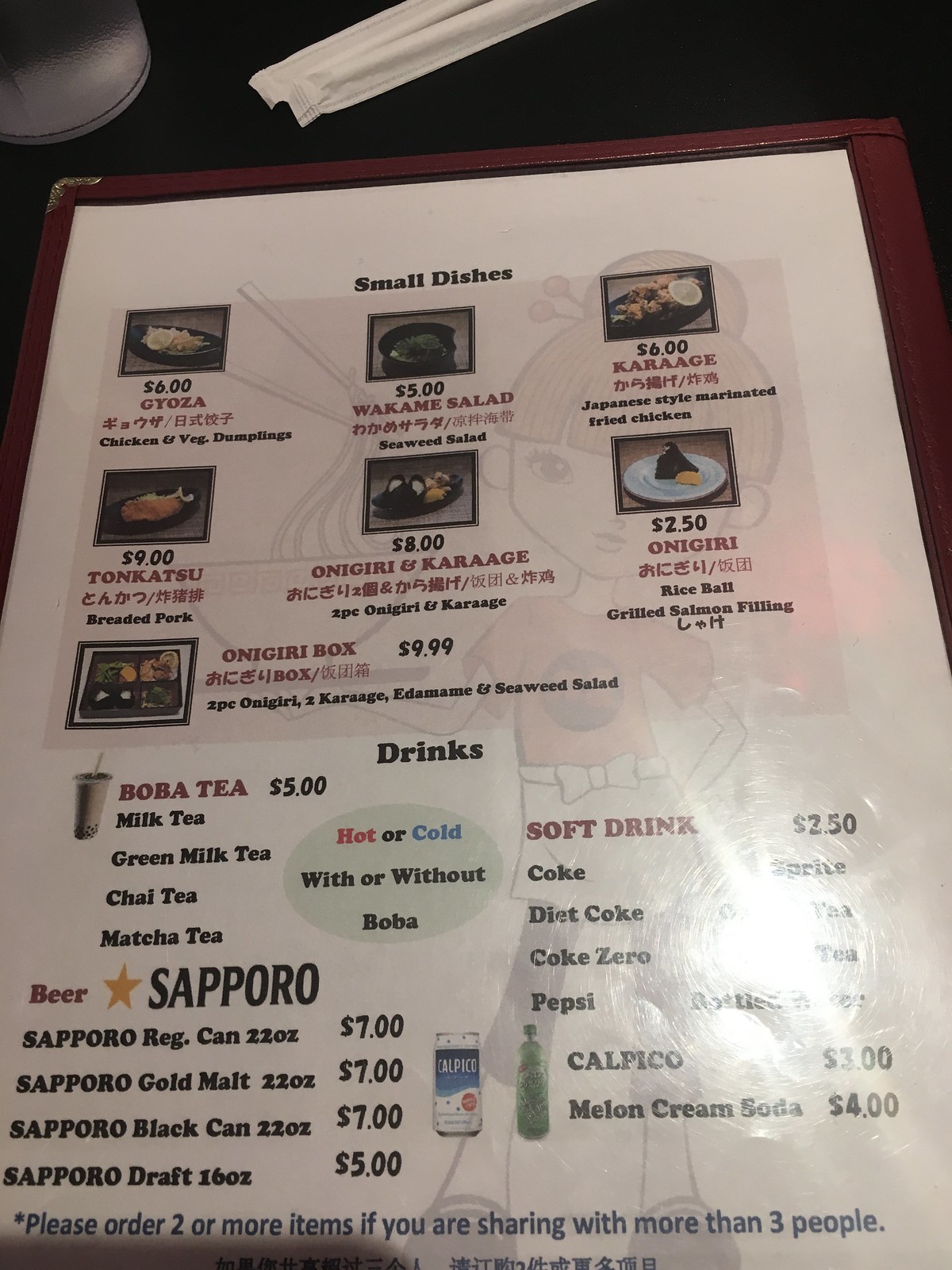In this vibrant color photograph of a restaurant menu, the detail brings the scene to life with rich descriptions. The menu lies open on a black tabletop, with the bottom edge of a cup or glass visible across the top of the image. Two straws in their white paper sleeves are angled diagonally from the middle top border toward the left, partially seen. The menu itself is housed in a faux leather cover, burgundy in color, accented with metal corner reinforcements, enveloping clear plastic that allows for easy cleaning and reuse.

The overhead lights cast a bright glare off the bottom part of the photo, creating a sharp contrast. The upper portion of the menu features small dishes, each accompanied by photo illustrations and text in both English and Japanese. 

The first dish is gyoza, labeled as "Chicken and Vegetable Dumplings" and priced at $6, displaying a tray of dumplings in a small photograph. Following this is a $5 Wakame Salad also identified as seaweed salad, with a corresponding photo. Next is Karaage for $6, described as "Japanese style marinated fried chicken." 

On the next line, Tonkatsu appears at $9, also detailed in Japanese as breaded pork cutlet, accompanied by a photo of the dish plated. Onigiri and Karaage, mentioned in both languages, follows, though it isn't clearly described. Next, a $2.50 item, Onigiri, described as a rice ball with grilled salmon filling, makes an appearance. 

The final item in the small dishes section is an Onigiri Box, priced at $9.99, labeled as a special containing onigiri and karaage, edamame, and seaweed salad, essentially functioning as a bento box. 

Beneath the small dishes, the section for drinks begins. Notably, the menu features an anime-style illustration in the background, showcasing a waitress with her hair in a bun, clad in an apron, holding a steaming bowl of ramen with noodles and chopsticks in the air.

The drinks listed include various types of boba tea at $5, in flavors such as Milk Tea, Green Milk Tea, Chai Tea, and Matcha Tea, available hot or cold, with or without boba. The beer options consist of Sapporo brand: Regular Can (20+ ounces) at $7, Gold Malt at $7, Black Can at $7, and a confusingly priced Sapporo Draft listed as "$1.00 $5.00." A note encourages customers to order two or more items if sharing with more than three people.

The right column lists soft drinks, each priced at $2.50, including Coke, Diet Coke, Coke Zero, Pepsi, Sprite, and tea—though the latter is partially obscured by the glare. The bottom entries mention Calpico, a Japanese soft drink brand, and Melon Cream Soda, priced at $4.00.